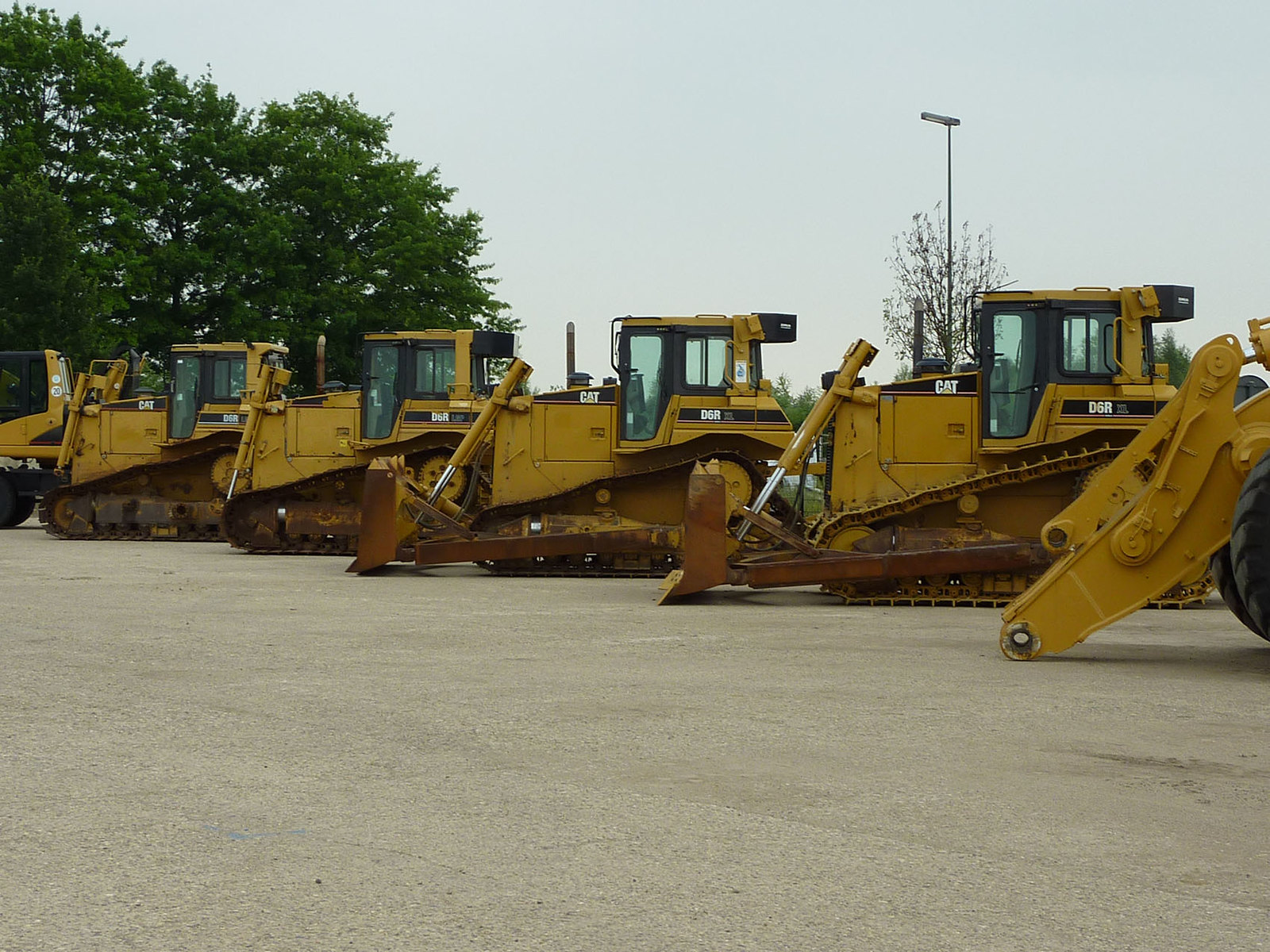The image is a color photograph showcasing a series of construction equipment lined up diagonally across the middle, extending towards the back left. The equipment includes a variety of yellow bulldozers and what appears to be the front of a JCB, all marked with the brand name "CAT" in white letters on a black background. The machinery is positioned side-on towards the viewer, with their fronts facing to the left, and they rest on tank-like tracks designed for traversing tough terrains. The leading machine, situated closest to the camera, partially reveals large black tires and a front attachment, possibly a digger or plow.

The foreground features a large expanse of concrete flooring in a sandy yellow hue, interspersed with dirt and dark brown speckles. To the left of the image, a large tree with dark green foliage reaches up to the left corner. On the right side, a street lamp stands vertically against a pale blue sky, which transitions to a slightly white shade near the treetops. The overall scene is captured during the daytime under clear skies, with a tree on the left and a partially leafless tree behind the street lamp on the right adding depth to the landscape.